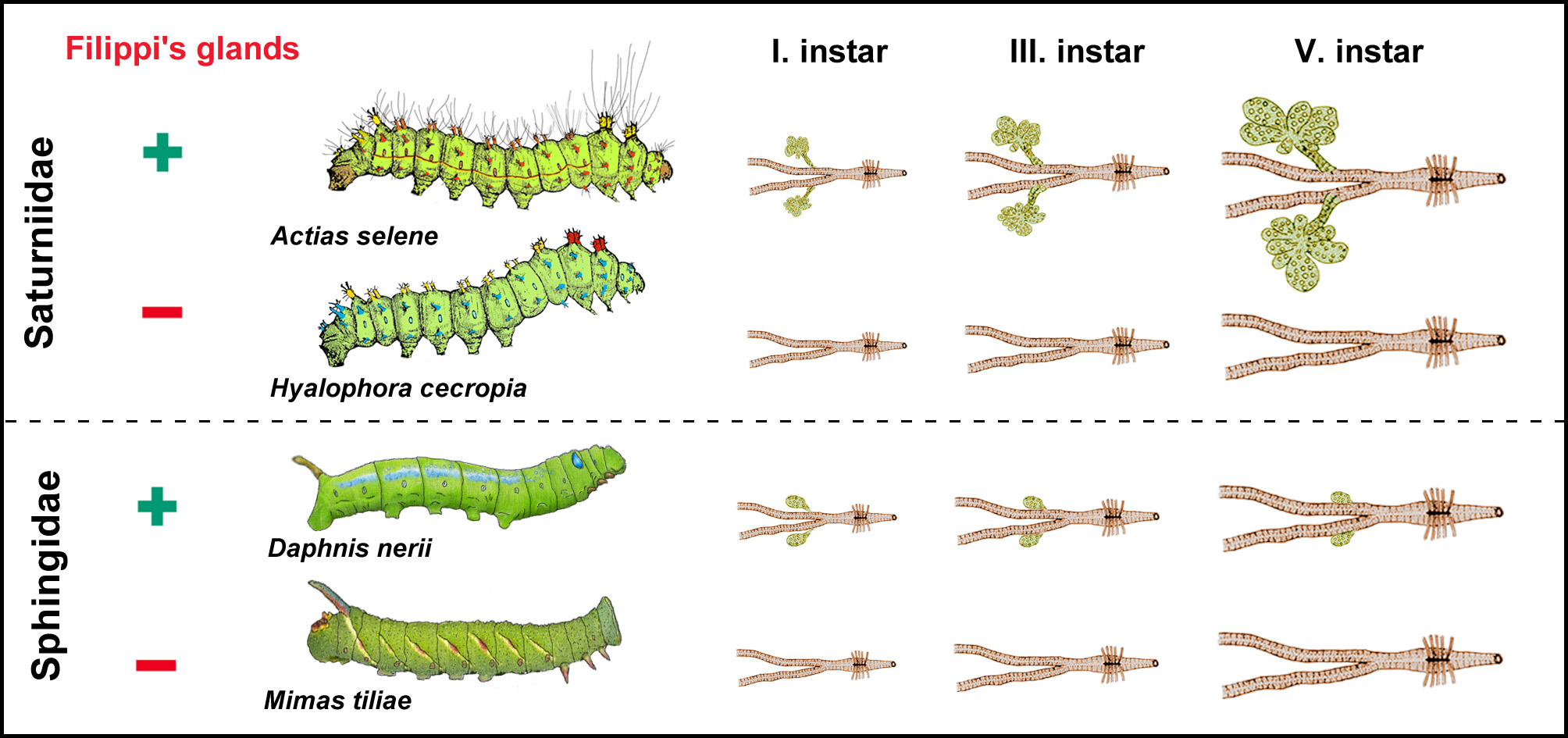This detailed color-scientific diagram depicts various types of caterpillars and their developmental stages, labeled according to specific parameters. At the top left corner, the words "Filippi's Glands" are prominently displayed. To the left, running vertically, are the family names "Sphingidae" and "Saturniidae." The diagram shows the caterpillars Actias selene and Hyalophora cecropia at the top half, divided by a dotted line from the bottom half, which features Daphnis nerii and Mimas tiliae. These caterpillars are presented in different postures, with Actias selene crawling rightwards towards three pieces of plant material, Hyalophora cecropia rearing up, and Daphnis nerii raising its head. The caterpillars, in varying shades of green, exhibit different textures—ranging from fuzzy and smooth to slimy and rough. On the right side of the diagram are graphical representations of developmental stages labeled "Instar 1," "Instar 3," and "Instar 5." The entire background is white, providing clear contrast to the colorful, detailed drawings of the caterpillars and plant matter.